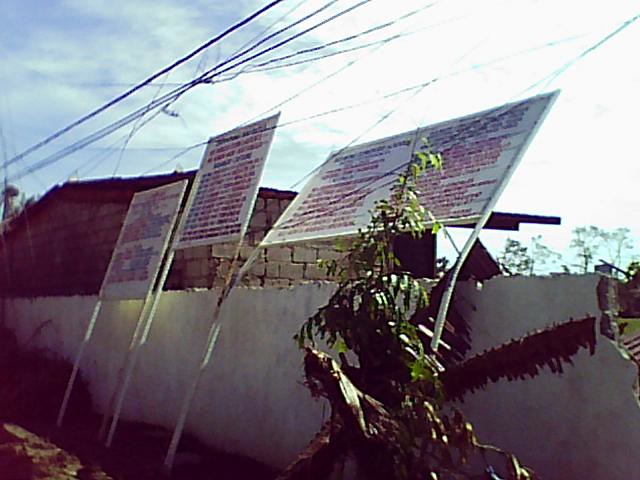The image depicts a scene of apparent wind damage set against a white flood wall. In the foreground, there are three signs with illegible lettering, each mounted on white poles. The first sign on the left is vertically oriented and supported by two poles; its lettering features red and blue text. The central sign mirrors this setup but is slightly taller. The last sign is horizontally oriented, suggesting it may have been tipped on its side due to the impact of strong winds, with all signs showing signs of leaning or bending. Above and around these signs, multiple electrical lines crisscross the clear blue daytime sky, some even draping across the signs themselves. A fallen palm tree lies in front of the signs, adding to the sense of wind damage. The background includes a partially visible concrete building with cinder block construction on the left and green shrubbery on the right. The ground in front of the signs appears partially muddy, hinting at recent adverse weather conditions.